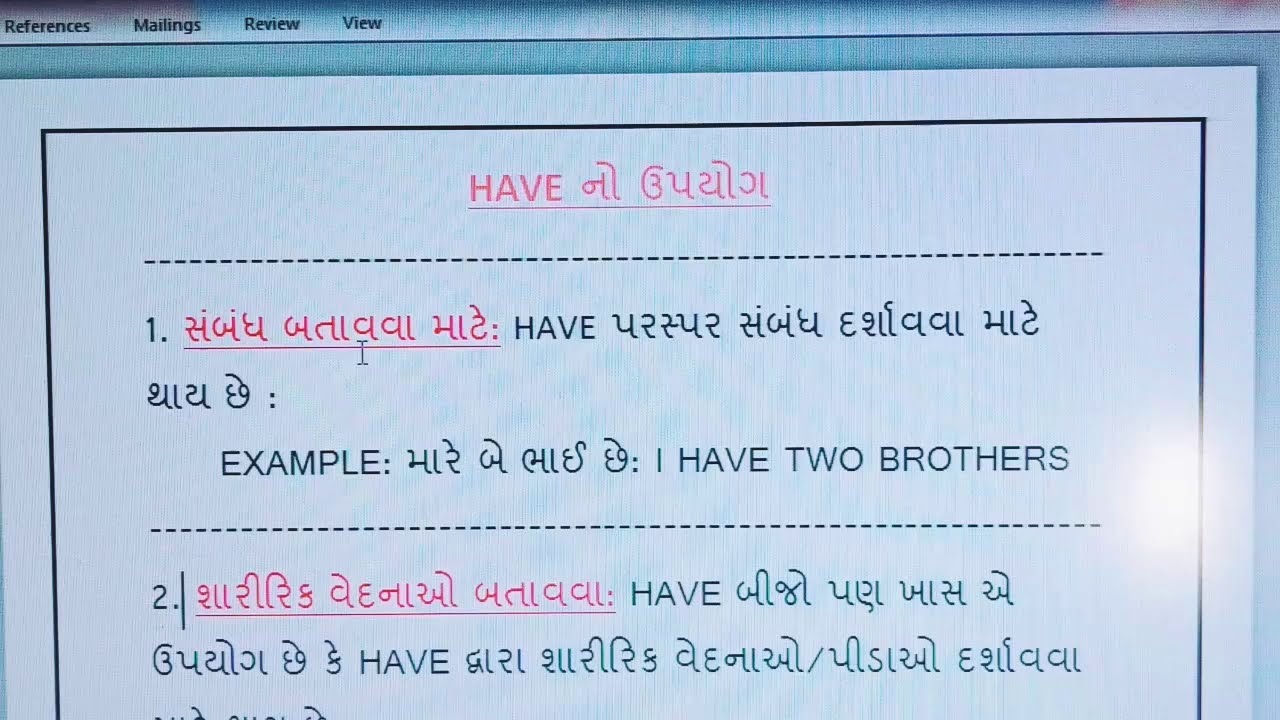The image depicts a photograph of a computer screen displaying a document. In the upper left corner, the words "References," "Mailings," "Review," and "View" are visible, each in black text. Beneath this menu, a black line is followed by a blue line that frames the entire document. The document itself has a black border around its edges.

At the top of the document, there is a section where the title "HAVE" appears in pink uppercase letters, followed by several characters from a foreign language. Below this title, a dotted line stretches across the page. Under the dotted line, the number "1" is present, succeeded by more pink foreign characters and the word "HAVE" again in uppercase. This is followed by additional foreign characters, a colon, and the word "EXAMPLE" in all uppercase black letters. Another colon leads to more foreign characters, followed by "I HAVE TWO BROTHERS" in black uppercase letters.

A dashed line separates the sections, and below this line, the document features the number "2," a period, a vertical bar, and more pink foreign characters, concluding with the word "HAVE" in black. Additional lines of foreign characters follow, and another line beneath this has "HAVE" centered, flanked by foreign characters. To the right side, there is a reflection of white light, indicating the image is an actual photograph of the screen rather than a direct screenshot. The overall content suggests it could be a language-learning document, potentially used for teaching English to speakers of another language or vice versa.